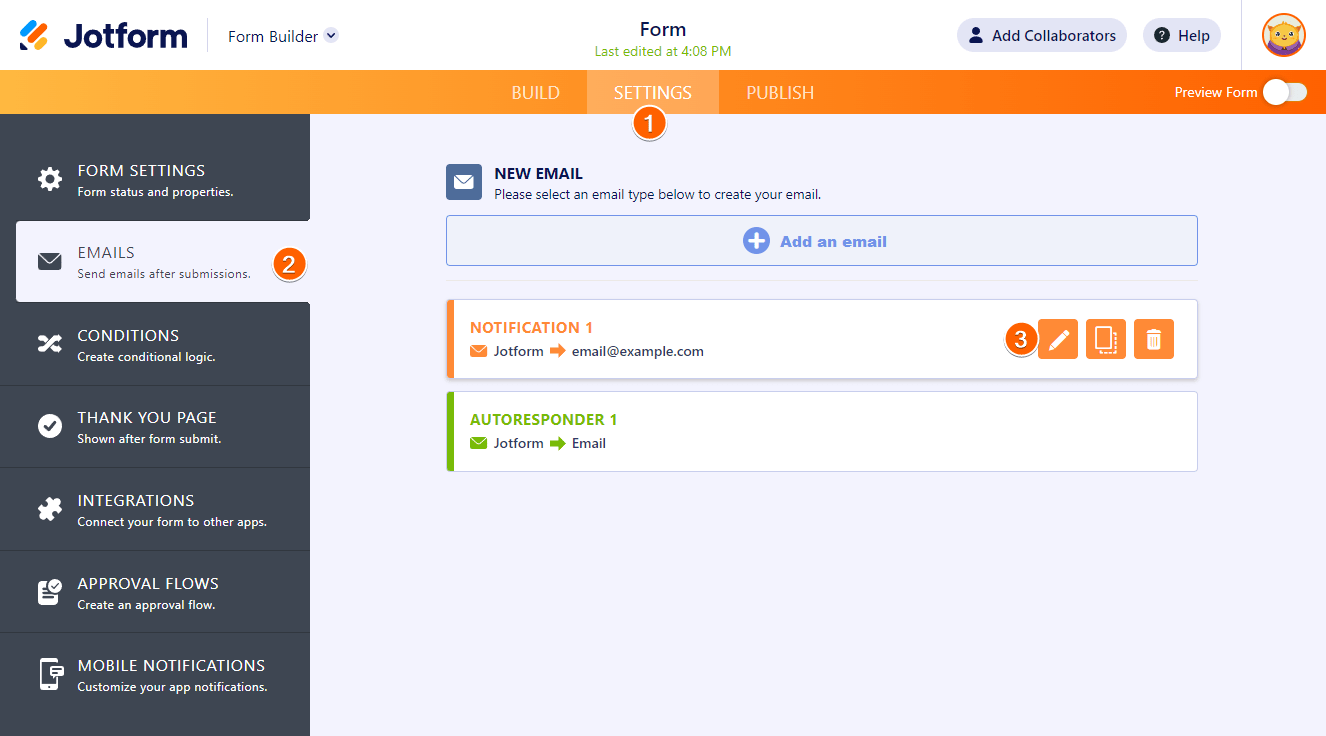This detailed screenshot captures the interface of a JotForm webpage. At the very top, a white banner spans across the screen, featuring the JotForm logo on the top left corner written in bold black letters. Next to it, in black letters, are the words "Form Builder," followed by a timestamp indicating the form was last edited at 4:08 PM, as well as options labeled "Add Collaborators" and "Help." Directly below the white banner, a gradient orange banner stretches from left to right, starting with a lighter shade of orange and transitioning to a darker shade. This banner contains navigation tabs labeled "Build," "Settings," and "Publish," with "Settings" being the currently selected tab, marked with a number "1" underneath it. Adjacent to these tabs are options reading "Preview Form" and a slider button, which is currently in the off position.

On the far left side, there is a vertical black menu displaying several options: "Form Settings," "Emails" (annotated with a number "2"), "Conditions," "Thank You Page," "Integrations," "Approval Flows," and "Mobile Notifications." Next to each menu item, a corresponding description provides functionality details.

The central part of the image focuses on email settings, highlighted by a prominent heading "New Email." The subheading instructs users to select an email type to create a new email, followed by a plus sign icon next to the text "Add an Email." Below this, two email notifications are listed: "Notification 1" linked to JotForm with an arrow pointing to the right, and an example email ("email@example.com") labeled with a number "3." Additionally, "Autoresponder 1" is listed with similar details - JotForm, an arrow to the right, and the displayed email.